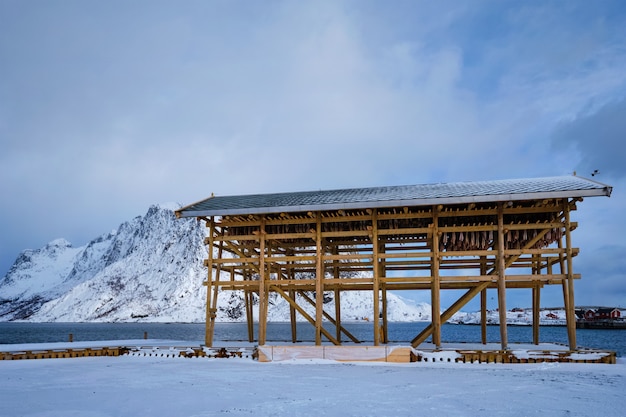The photograph captures a wintry, remote outdoor scene under daylight, utilizing natural light. The composition is square with no specific border or background. The top half of the image features a clear blue sky dotted with white clouds, while the lower part is blanketed in snow. Set against this backdrop, a wooden structure stands prominently at the center. The structure, appearing to be a shed or an unfinished building, is elevated on posts and completely open, devoid of walls, with cross beams crisscrossing throughout. The metal roof shelters an empty interior, save for some items, possibly fish, hanging from the rafters on the right side. 

In the background, towards the center left, a snow-covered rocky mountain rises, contributing to the cold ambiance. A body of still water, likely part of a river or bay, lies adjacent to this scenery, with some snow and ice visible along its edge. The foreground is entirely covered in snow, enhancing the wintry atmosphere. The overall appearance suggests a desolate, possibly northern location, evoking regions like Alaska or Nova Scotia. The site looks like a work in progress, anticipating further construction amidst the stark, frozen landscape.